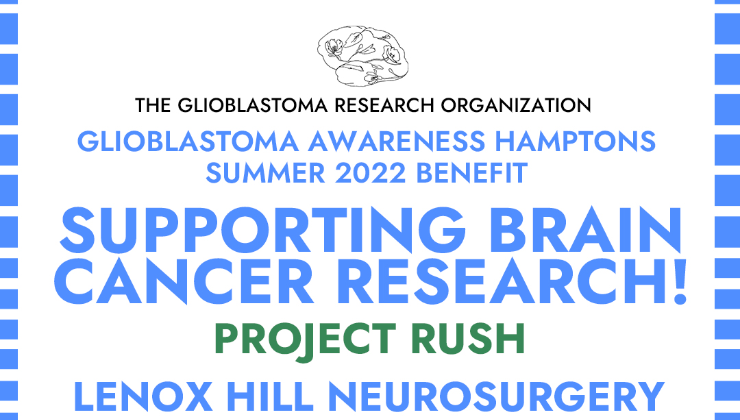The image being described is a horizontal rectangular poster or promotional banner with a white background. It features vertical blue rectangles along the right and left edges, resembling thick dashed lines that frame the image. At the top center, there is a black and white illustration that is ambiguous—it appears to be a brain with the intricate details of leaves and flowers interconnected within it, though it could also be interpreted as cells.

Below this illustration, in black capital letters, is the text "THE GLIOBLASTOMA RESEARCH ORGANIZATION." Beneath this, in blue capital letters matching the blue border, are the lines "GLIOBLASTOMA AWARENESS HAMPTONS" and "SUMMER 2022 BENEFIT," all centered horizontally. Following this, in much larger and bolder blue capital letters, are the lines, "SUPPORTING BRAIN CANCER RESEARCH!" Below this, in slightly smaller bold green capital letters, is the text "PROJECT RUSH." The bottom line of the image, also in blue capital letters, reads "LENOX HILL NEUROSURGERY." All text is aligned centrally on the white background, creating a visually structured and impactful announcement.